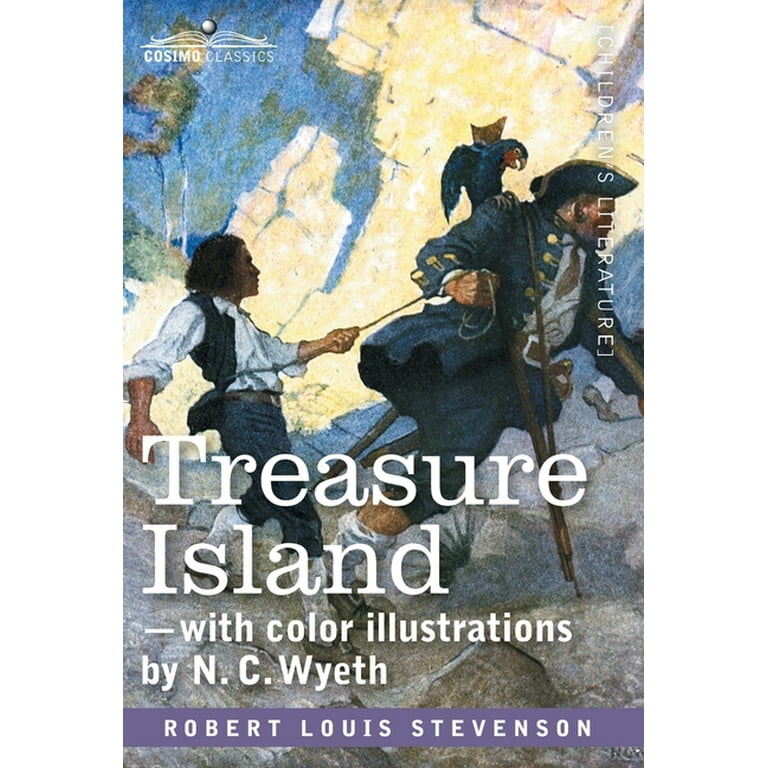This detailed cover of the children's book "Treasure Island" showcases a vivid illustration by N.C. Wyeth. Dominating the scene is a pirate with a peg leg, adorned in a suit overcoat with brass buttons, a pirate's hat, and a parrot perched on his shoulder. Accompanying him is a young man with dark hair, dressed in a white shirt, dark vest, blue or black pants, a gray belt, and white calf-length socks. Together, they appear to be climbing a rocky surface that transitions into a background featuring a white and yellow rock formation with green trees against a blue sky. The title "Treasure Island" is prominently displayed in white text, along with the note "with color illustrations by N.C. Wyeth," and at the bottom, it identifies the author "Robert Louis Stevenson" in white text on a purple banner. Additionally, the cover features the publisher’s mark, Cosimo Classics, in the top left corner with an open book logo.